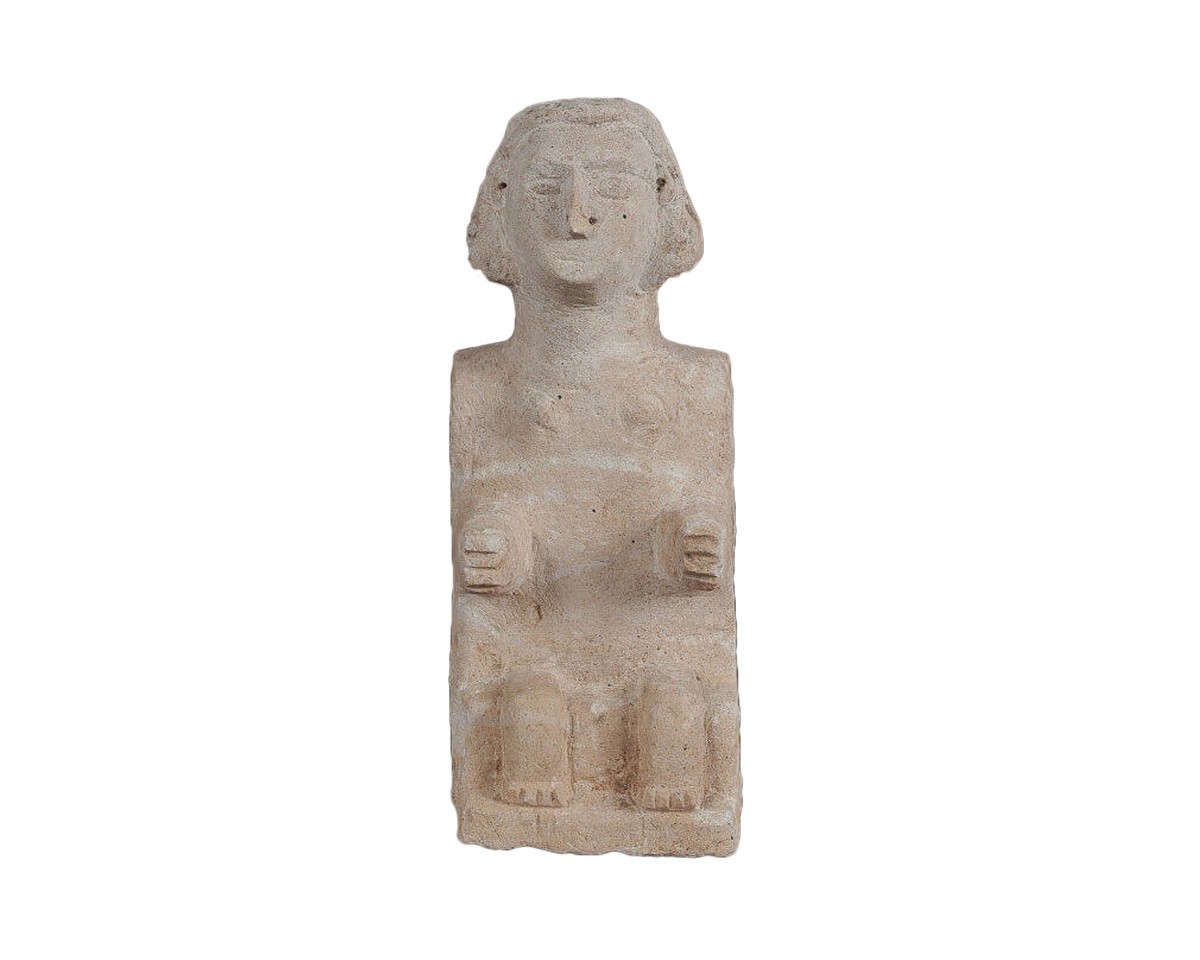This image features a primitive, tan-colored stone sculpture depicting a seated man. The sculpture's head is detailed with rudimentary features, including closed eyes, prominent eyebrows, a sculpted nose (with signs of slight damage), and a subtle line for the mouth. His hair appears styled in a bob cut. The proportions are notably childlike and imprecise, the body being a flat rectangular shape with minimal detail. Protruding mid-torso are two block-like representations of arms, each scored with three lines to suggest fingers. The legs, equally simplistic, are short rectangular blocks with similar markings to indicate toes, bent at the knees to rest on a square platform base. The sculpture evokes an archaic style, reminiscent of ancient and primitive cultures such as those of Easter Island or early ancient Egypt. The background of the image is plain white, focusing all attention on the statue itself.